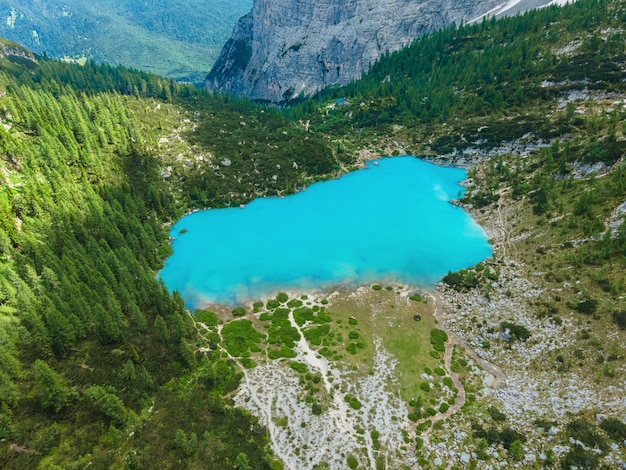The image captures a stunning outdoor scene that blurs the line between a photorealistic artwork and a high-quality photograph, perfect for hanging in a home. The central focus is a small pond, boasting remarkably clear, cyan-blue water that reflects the cloudless sky. This tranquil body of water is nestled within a valley surrounded by towering evergreen and pine trees. The left side of the image features taller, mature trees, while younger, shorter pines populate the right side. The foreground presents a mix of sandy, rocky terrain with patches of dirt and bushes. The background unveils a dramatic landscape of large, rocky mountains, completing the picturesque view. The composition suggests a vantage point either from a cliff or taken aerially at a high elevation, providing a breathtaking, expansive view of the natural beauty below. Daylight illuminates the scene, enhancing the vivid colors and textures that contribute to the overall serene and awe-inspiring atmosphere.